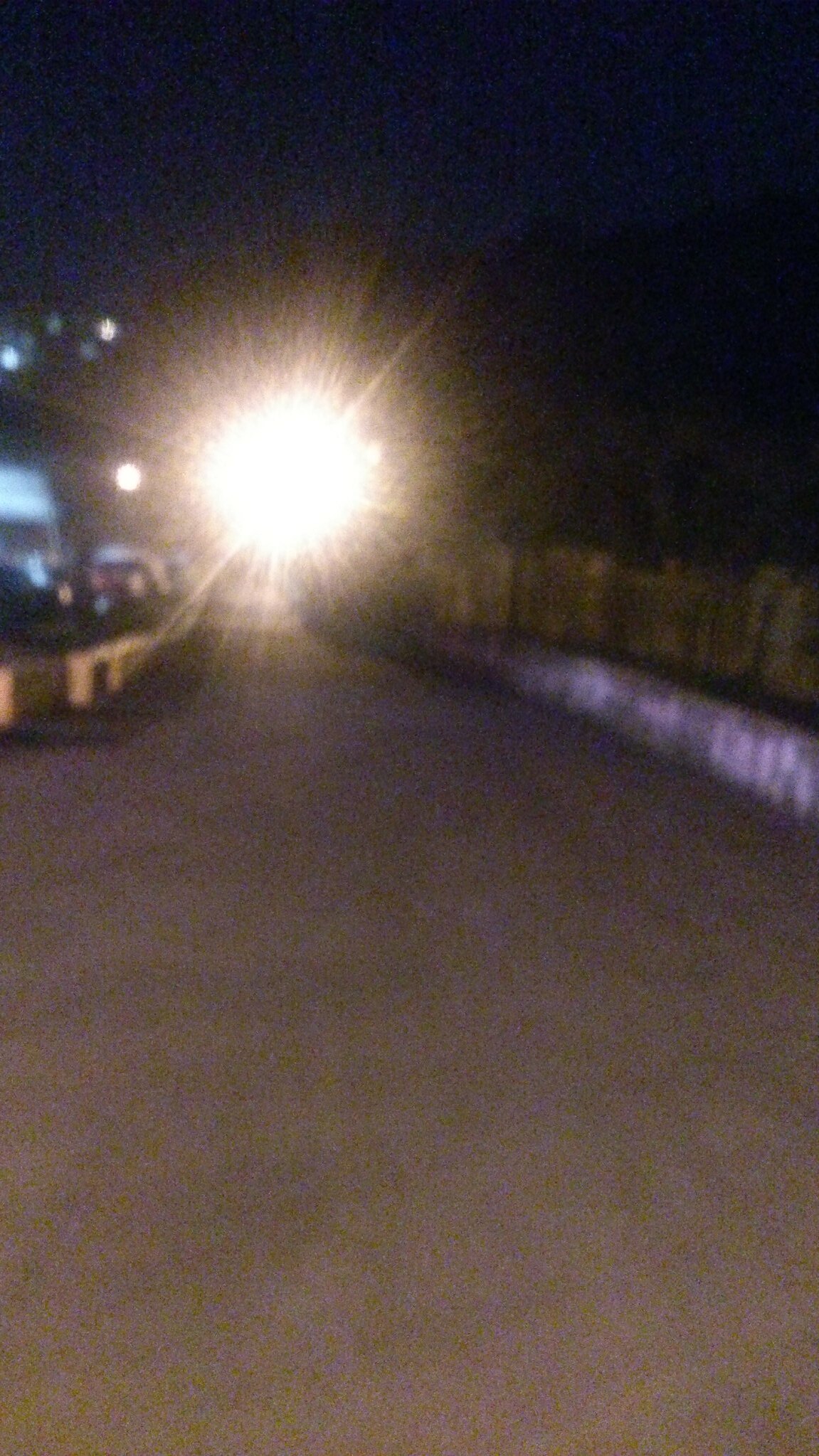A grainy, color photograph taken outdoors at night, possibly from a smartphone, features a tall portrait aspect accentuating its elongated nature. The upper third of the image is dominated by an intensely overexposed light source slightly to the left of center. The light creates haloing and streaks radiating outwards, obscuring its origin. 

In the foreground, a tarmac road widens before undulating into the distance. To the left, beneath the light's hot spot, the blurred outlines of parked vehicles are visible. On the right side, a tall curb runs along the road, appearing grey with possible pink spray paint. In the background, light brown fence panels are faintly visible, partially illuminated by the overexposed light. The top portion of the image is nearly black, with a hint of very dark bluish-purple tones suggesting the night sky.